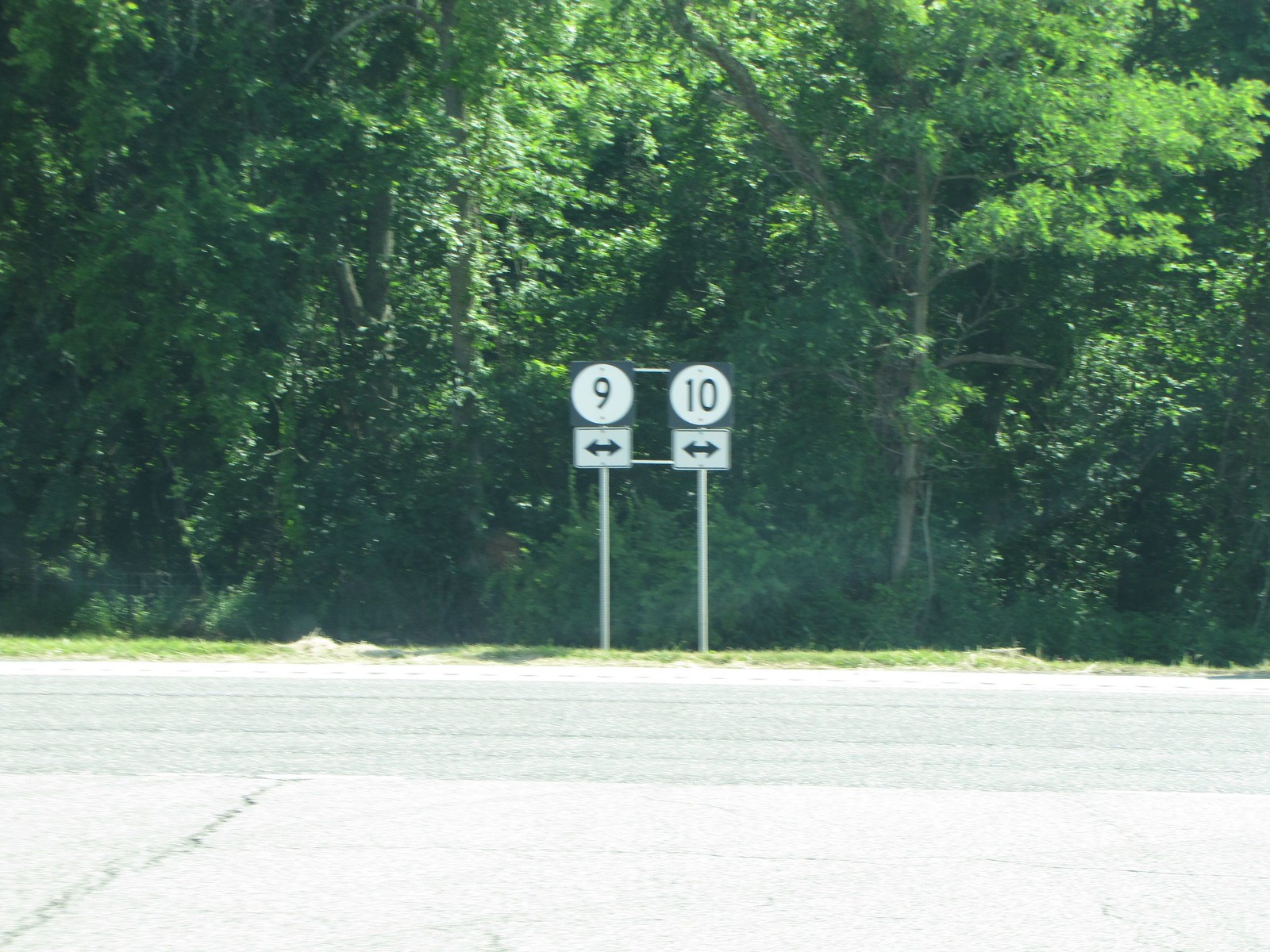This photograph captures the end of a street, featuring two prominent road signs mounted on a single silver metal frame. Each circular, white sign displays a black number—9 on the left and 10 on the right. Below each numbered sign, there is a rectangular sign with a two-headed black arrow pointing both left and right, indicating directional options. The signs are anchored into well-trimmed green grass, surrounded by lush trees with abundant green leaves and branches that fill the background. Sunlight can be seen reflecting off the leaves, highlighting the warm atmosphere of the area. In the foreground, a grayish-white cement road stretches out at the bottom of the image, further emphasizing the road's end. The background suggests a steep drop-off area, adding depth to the scene with its collection of green vines, bushes, and thickly wooded vegetation.